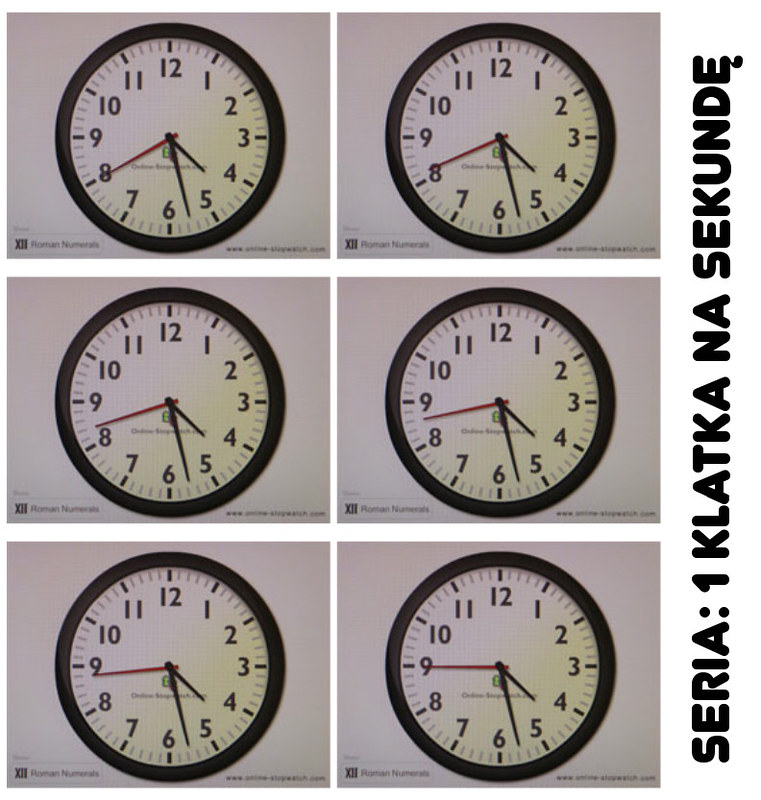The image depicts a gray wall adorned with six round black clocks. Each clock features a white face with black numerals and two black hands accompanied by a single red seconds hand. All six clocks are synchronized, indicating a time of approximately 4:27. Running vertically down the left side of the image, there is black lettering that reads "Serio 1 Klatka Nasekunde." The stark contrast between the elegant black clocks and the muted gray wall creates a visually striking display, highlighting the uniformity and precision of the timepieces.